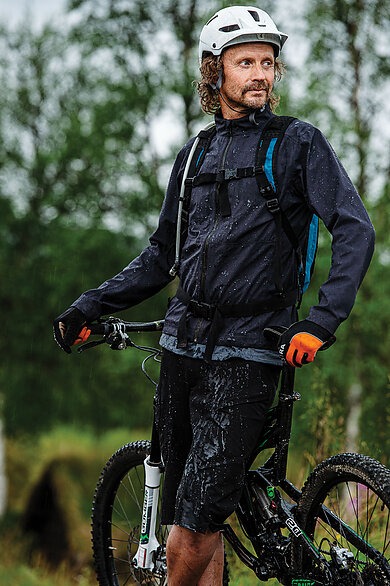In this image, we see a middle-aged white male cyclist standing in a blurred forest or garden area with lots of trees and greenery, and a clear sky. He has long, curly brown hair peeking out from under his white cycling helmet, which pairs with a beard and mustache. Dressed in dark waterproof rain gear consisting of a navy blue windshield jacket, black quarter pants, and black gloves with orange parts, he leans against his black bicycle. Both the man and bicycle are visibly wet, with water droplets noticeable even on the upper part of his jacket. The cyclist's backpack is secured with front buckles, and he gazes to his right, seemingly posing for a well-lit professional photoshoot. The image is slightly pixelated and noisy, but the focused subject contrasts sharply with the bokeh effect of the out-of-focus, richly colored forest and mountain background.